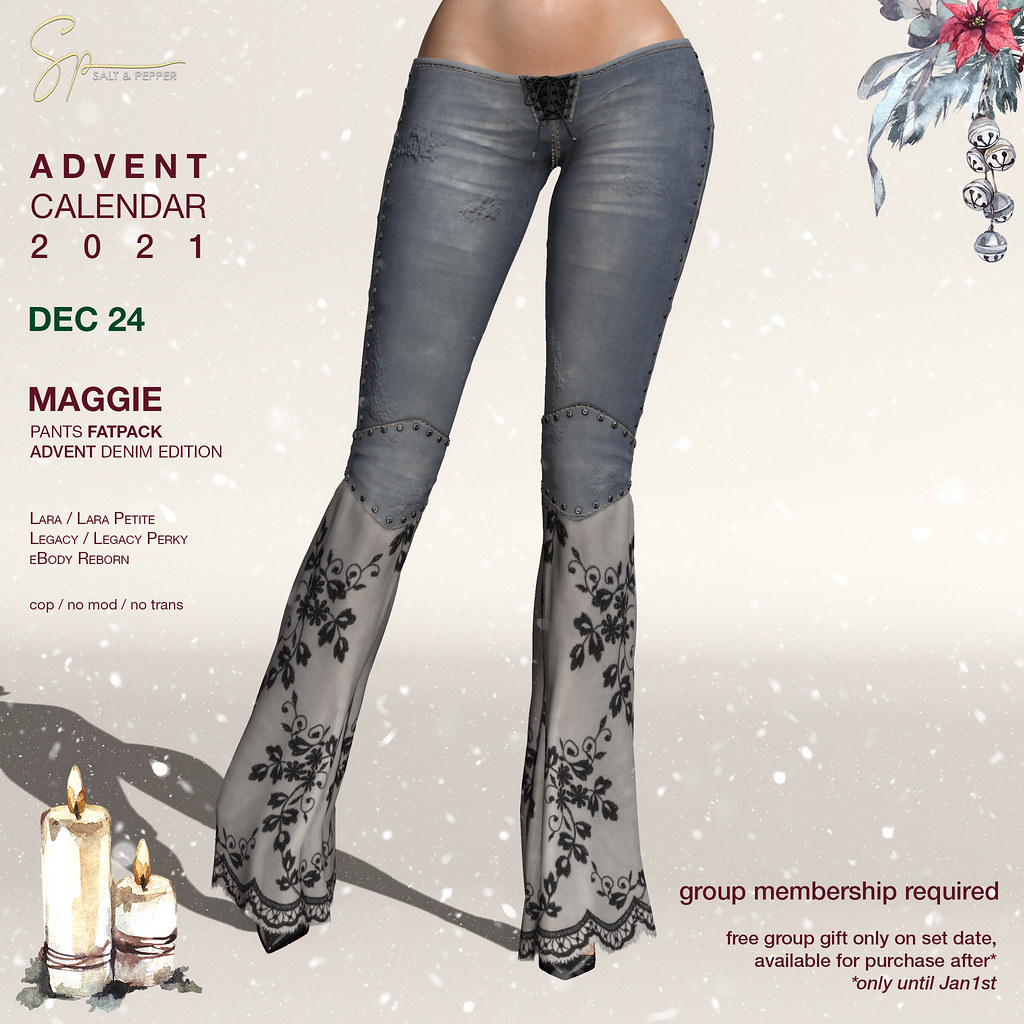This detailed advertisement flyer for jeans from the Advent Calendar 2021 prominently features an image of a female model's lower body, from the waist down. The model has dark skin and is wearing very low-cut bell-bottom jeans. The upper part of the jeans is classic denim, but from the knee down, the fabric transitions to a light gray color adorned with a black floral pattern. The jeans flare out at the bottom, and the model is stylishly accessorized with black pointy stiletto shoes. 

The design of the flyer is accented with a festive touch. In the lower left corner, two artistically drawn burning candles are visible, adding warmth to the visual theme. The background has a grayish tone with white specks, mimicking a snowy scene, and in the upper right corner, there is a pink poinsettia with jingle bells hanging beneath it. 

Text details on the flyer include essential information: "Group Membership Required. Free group gift only on set date. Available for purchase after until January 1st." Moreover, the top left corner reads "Advent Calendar 2021, December 24th, Maggie Pants Fat Pack, Advent Denim Edition," indicating the specific item and edition promoted. Additional text suggests compatibility for various body types: "Lara, Lara Petite, Legacy, Legacy Perky, and eBody Reborn," ensuring the product suits diverse preferences.